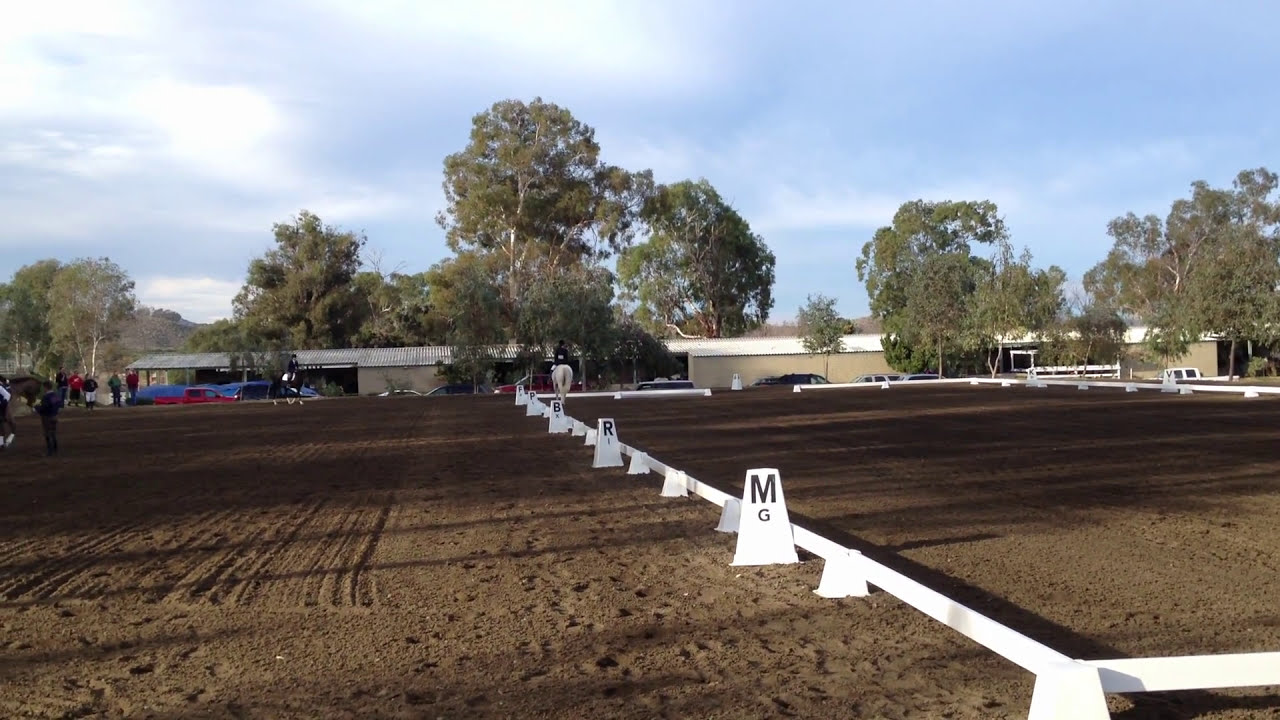This is a detailed outdoor photograph of a farm field, presenting two distinct sections divided by a boundary. The expansive ground is covered with brown, cultivated soil. On the left side of the image, the farm field lacks a boundary and features several people standing and a black horse with a rider, hinting at its use as a horse training area. On the right side, a fenced area is evident, constructed with white colored blocks and marking off a field, housing a white horse with a rider.

In the midst of the farm field, certain areas are marked with signs bearing black letters such as 'M,' 'R,' and 'G,' though their exact purpose remains unclear. Farther beyond the fields' borders, lush green trees form a backdrop along with some buildings, presumably barns or stables, accompanied by various vehicles including a distinguishable red truck on the left side. Above, the sky is painted a mixed blue with scattered white clouds, suggesting a clear, sunny day.

Additionally, a tan building with a white roof stands out in the background, with some cars parked in front. The overall color palette in the image includes white, brown, light green, dark green, blue, royal blue, black, and beige, showcasing the vibrant elements captured during the daytime.